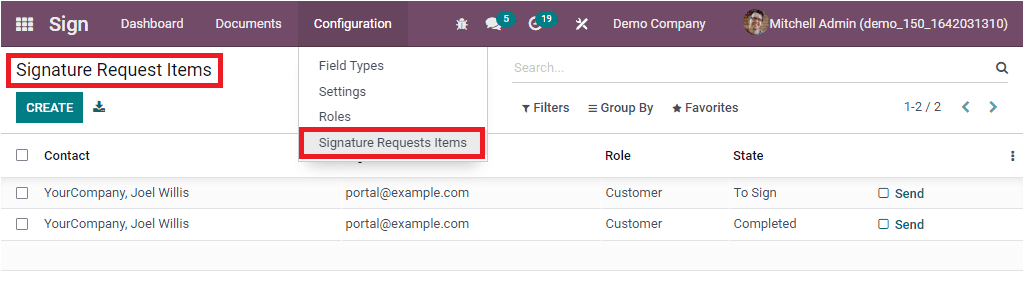The website interface features a distinct maroon navigation bar spanning across the top. At the center, the text "Demo Company" is prominently displayed, although there is no main title visible. Below this maroon bar is a white section labeled "Sign."

The main content area includes a structured layout with several sections. On the upper left is a menu box featuring circular icons and textual labels for "Dashboard," "Documents," "Configuration," and "Demo Company." There is also a mention of "Mitchell Administration" alongside a demo number.

A section titled "Signature Request Items" is bordered with a red outline, making it stand out. Adjacent to it is a green "Create" bar for generating new items. 

Under the "Configuration" section, there's a dropdown menu which includes options such as "Field Type Settings," "Roles," and "Signature Request Items," all similarly bordered with red.

Lastly, there is a section labeled "Contact," where users can toggle options. The contact details displayed include "Your Company Joel Willis" twice. Two circular green icons, one with the number 19 and another with the number 5, possibly indicate message notifications.

Additional functionalities include filters like "Group By," "Favorites," and a white search bar to facilitate easy navigation and search.